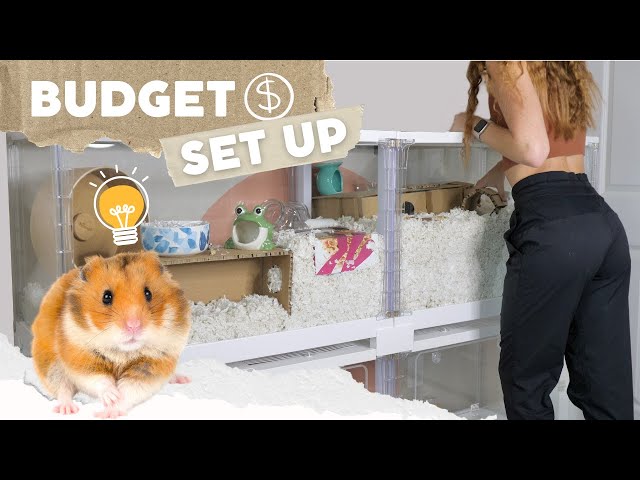In this image, a striking scene unfolds where a cute brown and white hamster with big brown eyes stands prominently under a cartoon lightbulb glowing with yellow and orange hues, suggesting an idea. The hamster is depicted in the foreground, flanked by a green stuffed frog, a blue and white Kleenex box, and several containers filled with shredded white paper, likely meant for nesting. The background features items essential for pet care, including a running wheel and various hiding spaces, hinting at a "budget setup" for owning a hamster or gerbil.

To the right of the hamster stands a young, shapely woman, her back turned to the camera. She has long brown hair cascading down to her upper back, beneath which she wears a sleeveless brown top that reveals her bare midriff, and black jogger pants. Her fair-skinned left wrist sports a silver watch with a black face. She appears to be engaged with the containers, possibly sifting through the shredded paper, indicative of preparing or shopping for pet supplies. The black bands at the top and bottom of the image frame the scene, accentuating the focus on both the hamster and the woman's engrossed action, suggesting an advertisement geared towards prospective hamster or gerbil owners.